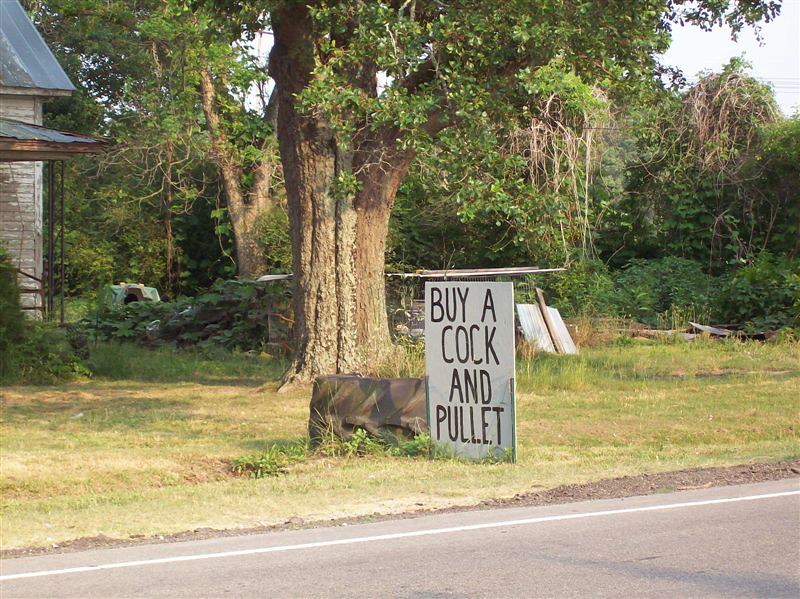This square color photograph captures a rural scene in the United States during summer. In the foreground, a mowed grassy area borders a strip of road running from the bottom left to the bottom right of the image. Dense foliage and beautiful oak trees form the backdrop, with a glimpse of a wooden-framed house topped with a blue slate roof visible on the left. To the right of the house, there appears to be a stone barbecue pit and a distinctive dark gray rock, possibly metallic with wavy lines, marking the edge of the property. A prominent feature is a white vertical rectangular sign near the center of the image, with black lettering that reads, "Buy a cock and pullet" – a humorous play on the words "cock" (a male rooster) and "pullet" (a young female chicken).